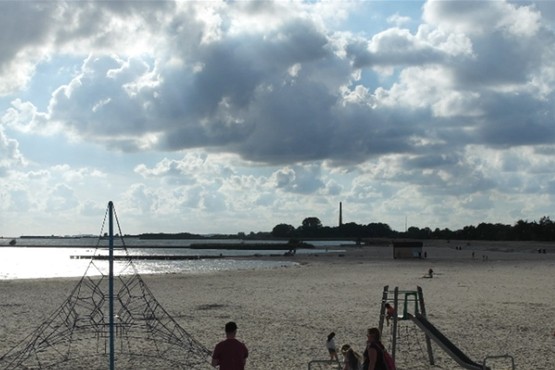The image depicts a bustling beach scene under a sky filled with gray clouds, through which rays of sunlight peek. To the left, the sun is partially obscured by clouds, casting a subtle shadow over the beach. On the left side of the image stands a playground with a jungle gym-like structure composed of a long pole and an intricate network of ropes for climbing. Adjacent to the jungle gym, to the right, there’s a children's slide, with a child seen at its top. In the foreground, five people are distinctly visible—comprised of three children, a man, and a woman who appears to be wearing a backpack. Scattered throughout the beach are additional small figures, creating a sense of liveliness. In the distance, near the horizon, stands a tall, mysterious tower and a small hut-like structure. Stretching from the middle to the right side of the horizon is a tree line that borders the sandy shore. On the left side, the vast expanse of water gleams under the sunlight.